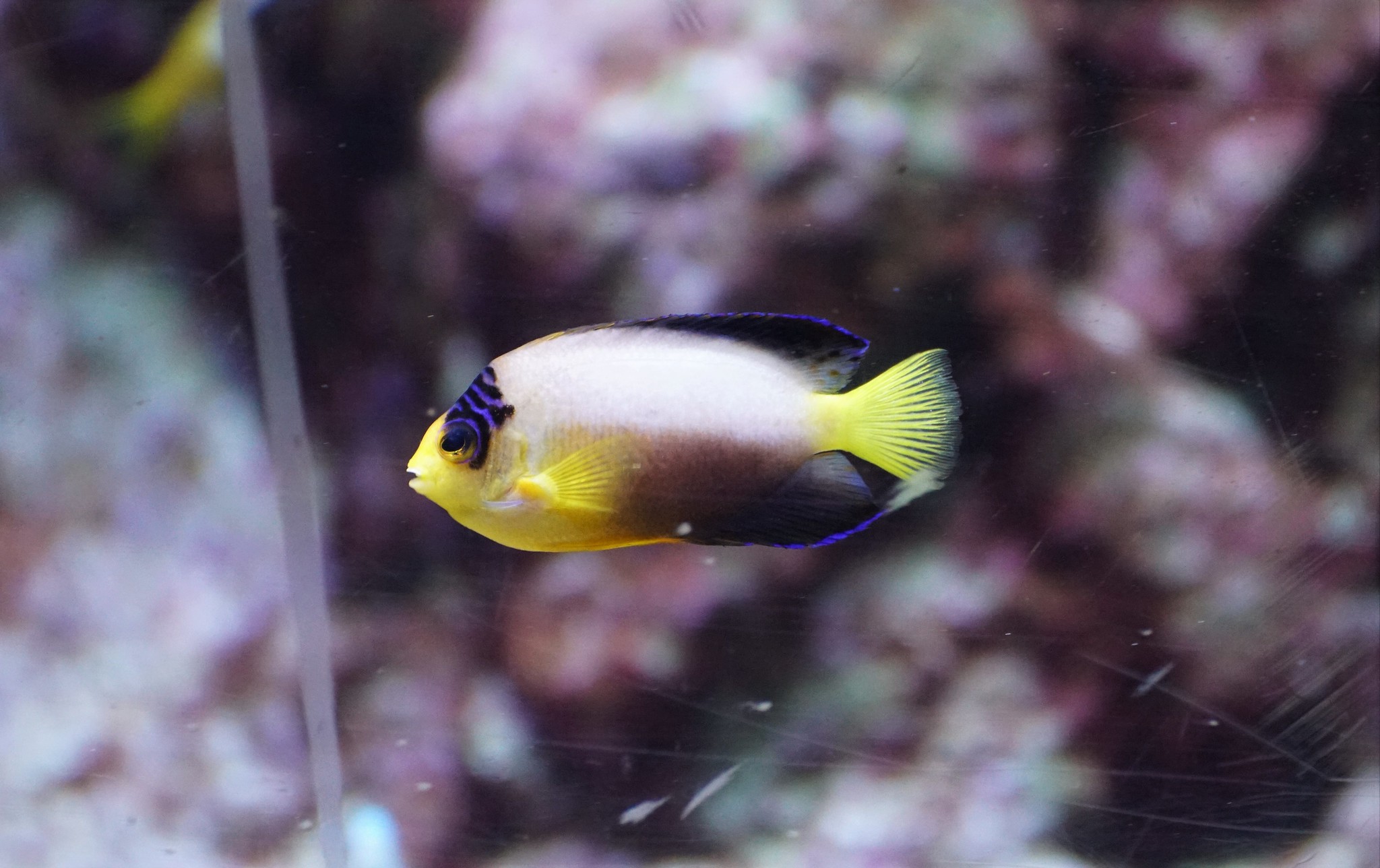The photograph captures a single teardrop-shaped fish in an aquarium, positioned centrally and viewed from the side with its face pointing left and tail to the right. The fish features a distinctly bright yellow tail fin edged with black, while its top and bottom fins are black trimmed with bright blue. Its swimming fins on the sides are yellow. The fish's body showcases a gradient, with the top half being white and transitioning to brown on the back lower half, while the front lower half is yellow. Surrounding its black eye, a striking black and blue leopard-style pattern is noticeable. The image, taken through aquarium glass, reveals various smudges and scratches, with a blurry background hinting at coral or artificial elements in reds, greens, and whites.